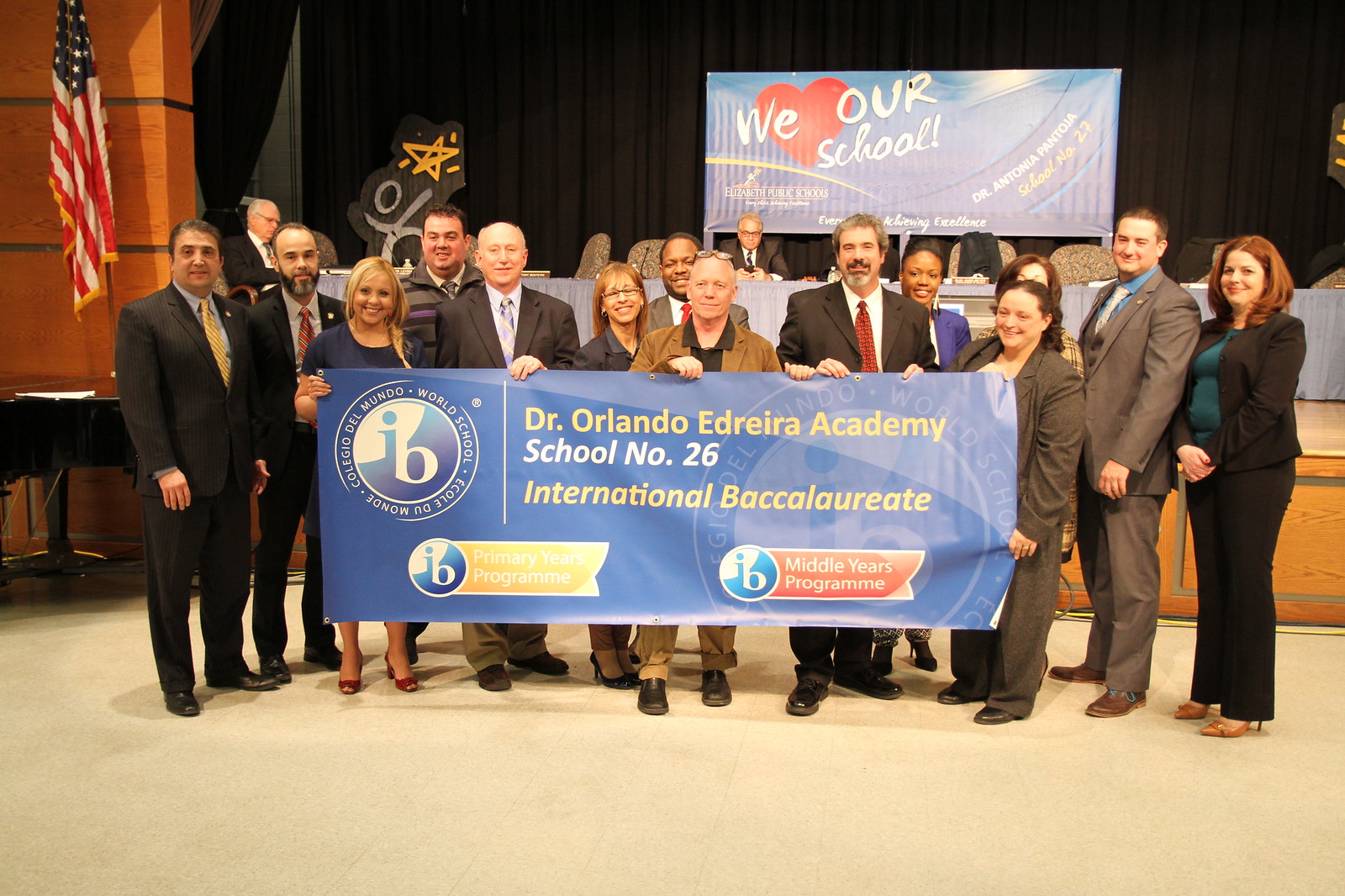In this detailed image of an academic event, a diverse group of over a dozen men and women is standing on a cream-colored floor, facing forward. The delegates, representing various countries and ethnicities and spanning different age groups, are dressed in formal attire; men in black suits with white shirts and ties, and women in either blazers and pants or dresses. They hold a large, rectangular, blue banner that reads: "Dr. Orlando Edevarera Academy, School NO 26, International Bachelorette, Middle Years Program, Primary Years Program." The banner features a logo with "IB" at the center, encircled by the phrases "Collegio del Mundo," "World School," and "École du Monde."

Behind the group is a stage with a long table, topped with chairs, water bottles, and other items. Two men in black suits, white shirts, and black ties are seated at the table; one of them, clean-shaven and wearing glasses, is looking at his mobile phone. The backdrop of the stage features a black curtain with a prominent blue sign adorned with a large red heart and the words, "We Love Our School," indicating "Elizabeth Public Schools" and showcasing a partially visible school motto, likely "Every Child Achieving Excellence." Additional details include another banner with "Dr. Antonia Pantoja School Number 27," a design or graffiti featuring stars and images, an American flag to the left, and a glimpse of an orange-colored wall with a desk and some papers in the background.